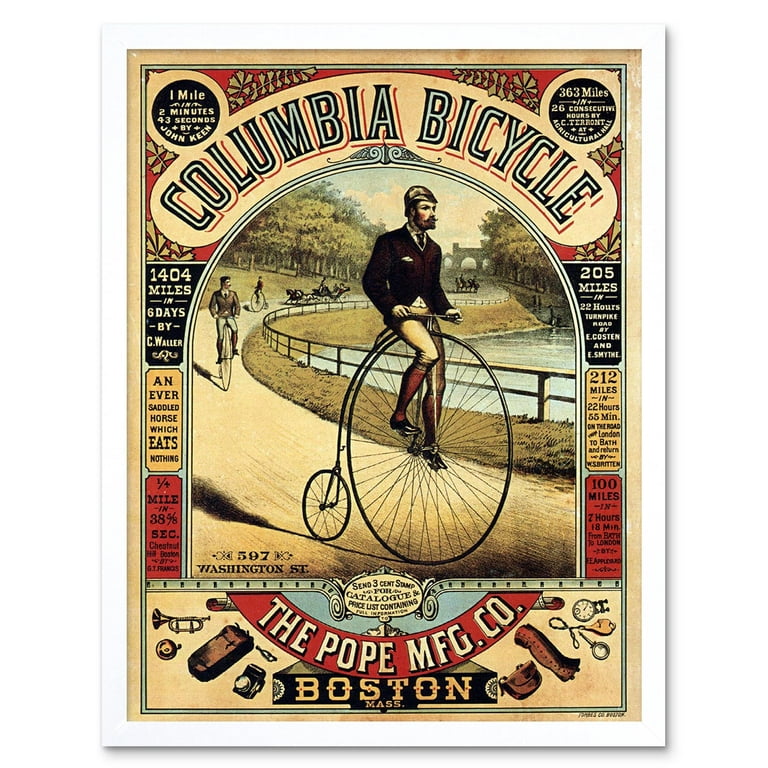This image appears to be an old-fashioned advertisement for the Columbia Bicycle, resembling a painting or a lithograph from the 1800s. Dominating the scene is a sharply dressed man riding a distinctive high-wheel bicycle, known for its very large front wheel and much smaller rear wheel. He wears a suit jacket, cravat, cap, and tall socks, with a handlebar mustache completing his look. In the background, other individuals are also depicted on similar bicycles. Surrounding the main illustration, the poster is filled with various text and details, including accomplishments and features of the bicycle, such as "1,404 miles in six days by C. Walter," and "one quarter mile in 33 and 58 seconds." The text, reminiscent of poker cards or circus-style fonts, promotes the durability and uniqueness of the bicycle, referring to it as "an ever saddled horse which eats nothing." The ad is decorated with several illustrations of different items produced by the company, including a watch, keys, boots, a trumpet, and drums, all in muted colors like browns, beiges, and muted reds. At the bottom, it states "The Pope Manufacturing Company, 597 Washington Street, Boston, Mass," surrounded by various product illustrations.